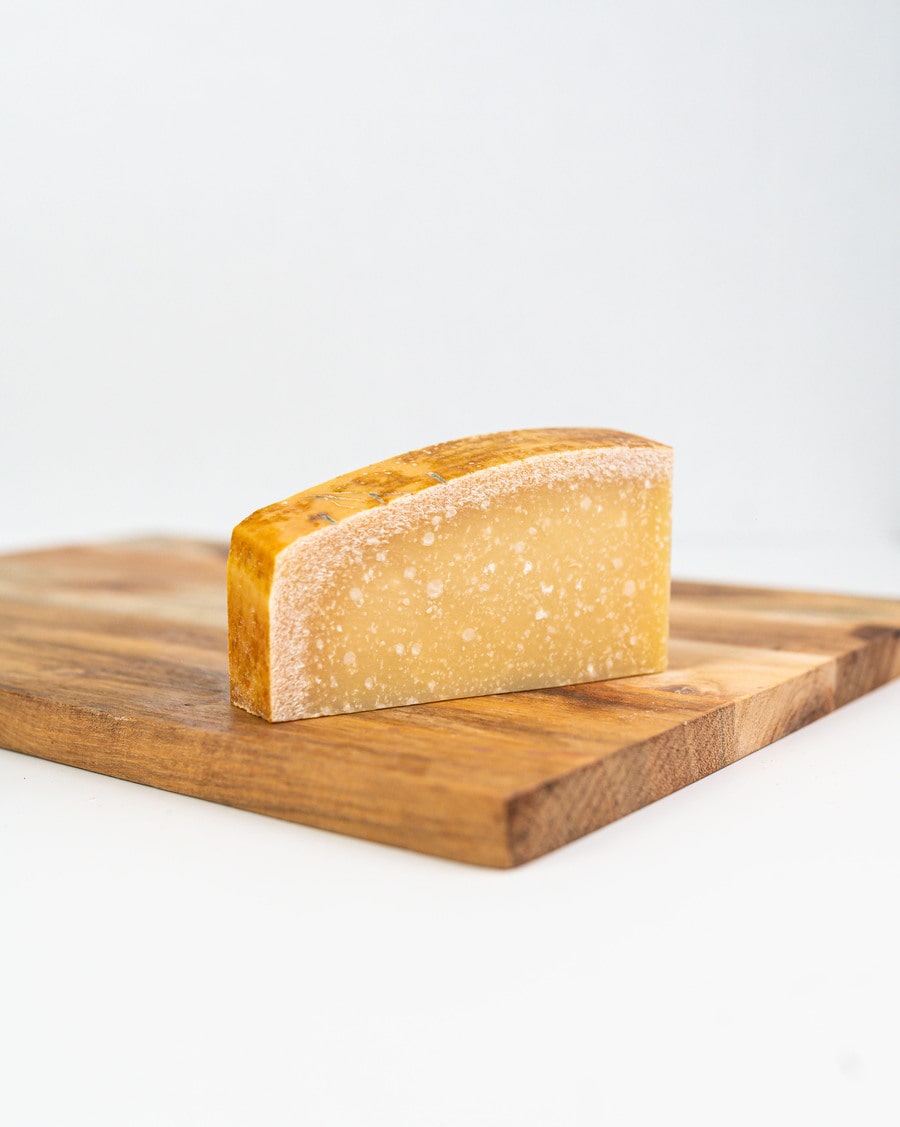The photograph features a rectangular, medium-tone wooden cutting board with natural wood grain variations, placed on a white countertop that transitions to light gray at the top. The central focus is a chunk of cheese positioned on the cutting board, showcasing its rustic appeal. The cheese has a rough, dark yellow rind with brown patches and a snow-like white mold pattern near the surface. The inner cheese is a pale yellow, resembling a hard cheese such as Parmesan. The scene is minimalistic, with no other items or utensils visible, emphasizing the cheese's texture and the cutting board's simple, natural aesthetic.